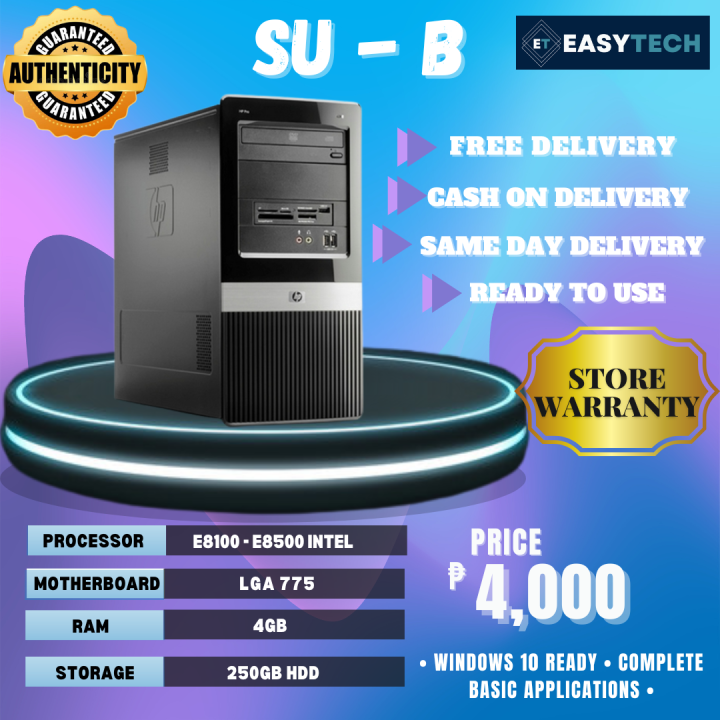The image features an HP branded computer tower prominently displayed. The upper left corner showcases a "Guaranteed Authenticity" stamp, while the center right highlights a "Star Warranty." The top right features the name "EasyTech," suggesting the retailer of the device. The top center bears the label "SU-B" and lists several key selling points including "Free Delivery," "Cash on Delivery," "Same Day Delivery," and "Ready to Use."

The HP computer tower itself is standard in design. At the upper section, it houses a DVD/CD drive. Below that, a variety of ports are available, including slots for different memory cartridges and external devices, a microphone jack, an audio jack, and two USB ports. Inside, the tower is equipped with an E8-100 to E8-500 Intel processor and a motherboard designated as LGA-775. It boasts 4GB of RAM and 250GB of HDD storage.

The device is listed at a price of 4000, although the exact currency is unspecified. The description notes that the computer is "Windows 10 Ready" and comes pre-installed with basic applications.